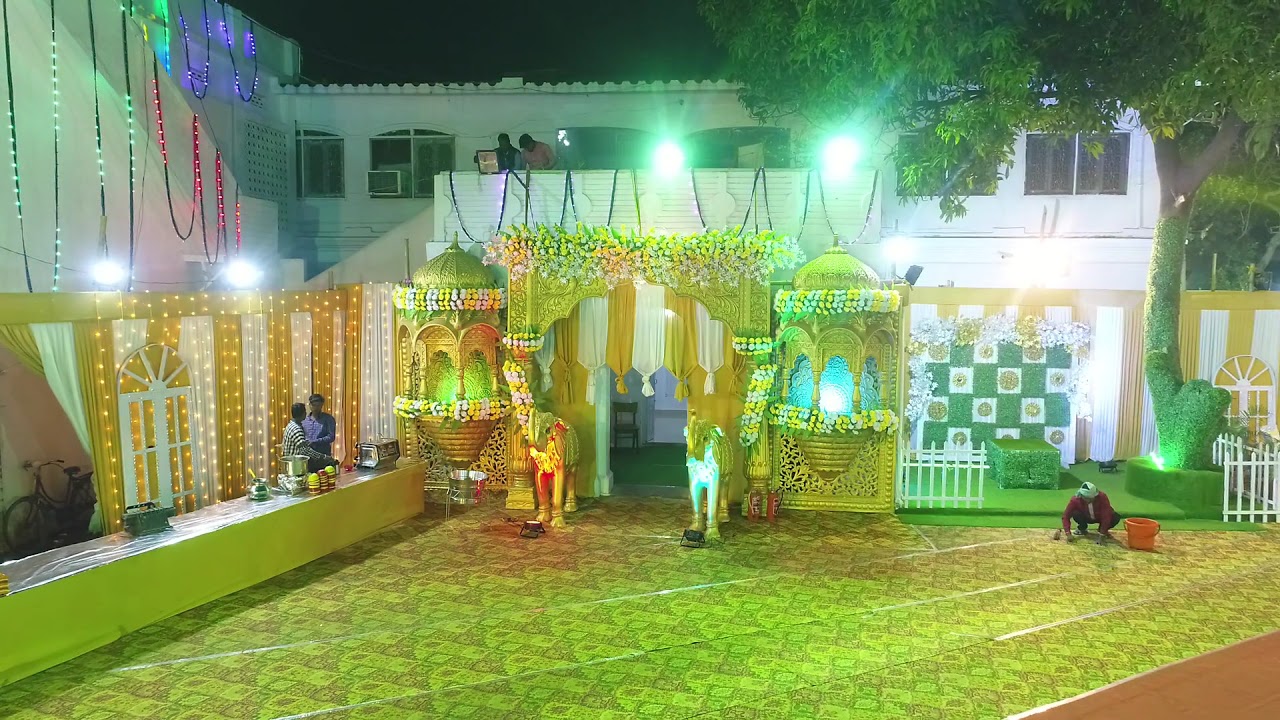This nighttime outdoor photograph showcases a vibrant Indian-themed courtyard, suggesting preparations for a special event. Dominating the background is a tall, silver-white building with gold trim and balconies, illuminated by two bright spotlights that obscure the clear view of the two individuals present there. Beneath these balconies is an ornately decorated archway adorned with white and gold banners, hanging curtains, and vibrant yellow flowers. Flanking this archway are intricately crafted elephant statues, one red and gold, the other white and gold. The left side of the image features a long row of tables with utensils and two people, likely setting up for a banquet. The right side captures a person crouched on the floor, seemingly installing an ornate gold carpet. Adding to the vivid scene are string lights, lush plants and trees, and a greenish carpeted section with a small brown area in the bottom right corner. The color palette of the scene includes rich golds, yellows, whites, reds, blues, greens, blacks, and orangish hues, bringing the festive ambiance to life.